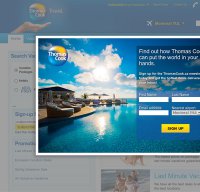In the small and distant screenshot, a Caucasian hand holds a circular object at the top. The object is adorned with a band of gold and yellow, featuring white text starting with "sun" and the letter "C" on a stark blue background, accented with cyan at the lower left. Superimposed on the circle is a rectangular image of a sky filled with white and pink-tinged clouds, underlined by dark blue and cyan strands.

Beneath these clouds is a resort scene. The resort includes dark grey-topped buildings with tan sides, resembling open shacks. On the right, there are several faded and blurred umbrellas, possibly white and blue, alongside leather chairs lining the edge of a tan stone pathway. Adjacent to this is crystal blue water that mirrors the sunlight, extending from a pier that accommodates the umbrellas.

In white text on the right, the words "find out how Thomas," cut off and followed by "C.O.," imply the potential of putting "the world in your hands." This text rests against a semi-transparent box, blending with the white clouds and blue sky behind it. Multiple other rectangles within this box have blurry white text, where the first appears to prompt for a first name, the next for a last name, and a new line for an email address. To the right, red text suggests selecting a destination. A yellow rectangle features black text, possibly reading "UAF" on the right and a barely discernible "EPO something H" on the left.

Overall, the image captures an idyllic resort setting underscored by promotional text encouraging a personalized experience.